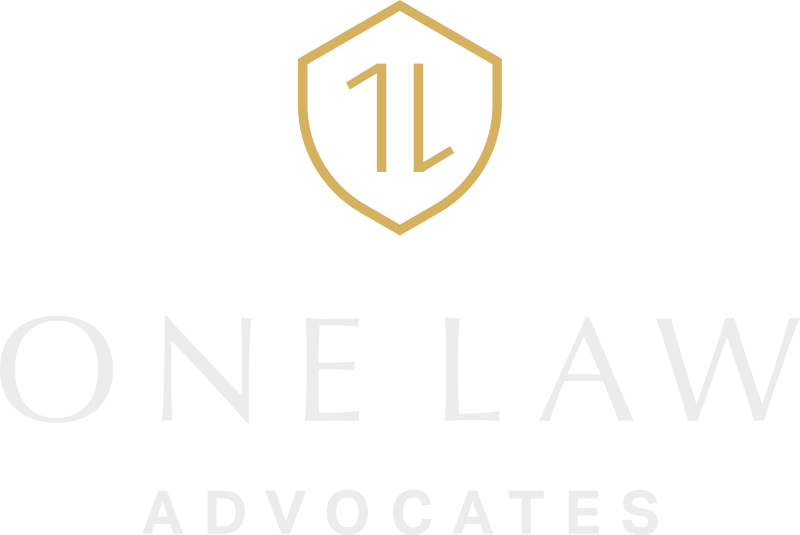The image features a minimalist advertisement for a law firm against a white background. Dominating the upper center of the image is a distinct gold-outlined badge or shield with curved edges, giving it a unique, rounded triangular appearance. Within this shield, there are two gold symbols: a number one on the left, and an upside-down number one on the right, resembling a slanted L. Beneath the shield, in large, light gray capital letters, is the firm's name, "ONE LAW," followed by "ADVOCATES" in smaller capital letters of the same light gray hue. The simplicity and elegance of the logo and text create an authoritative and professional look, seamlessly blending into the stark white background.